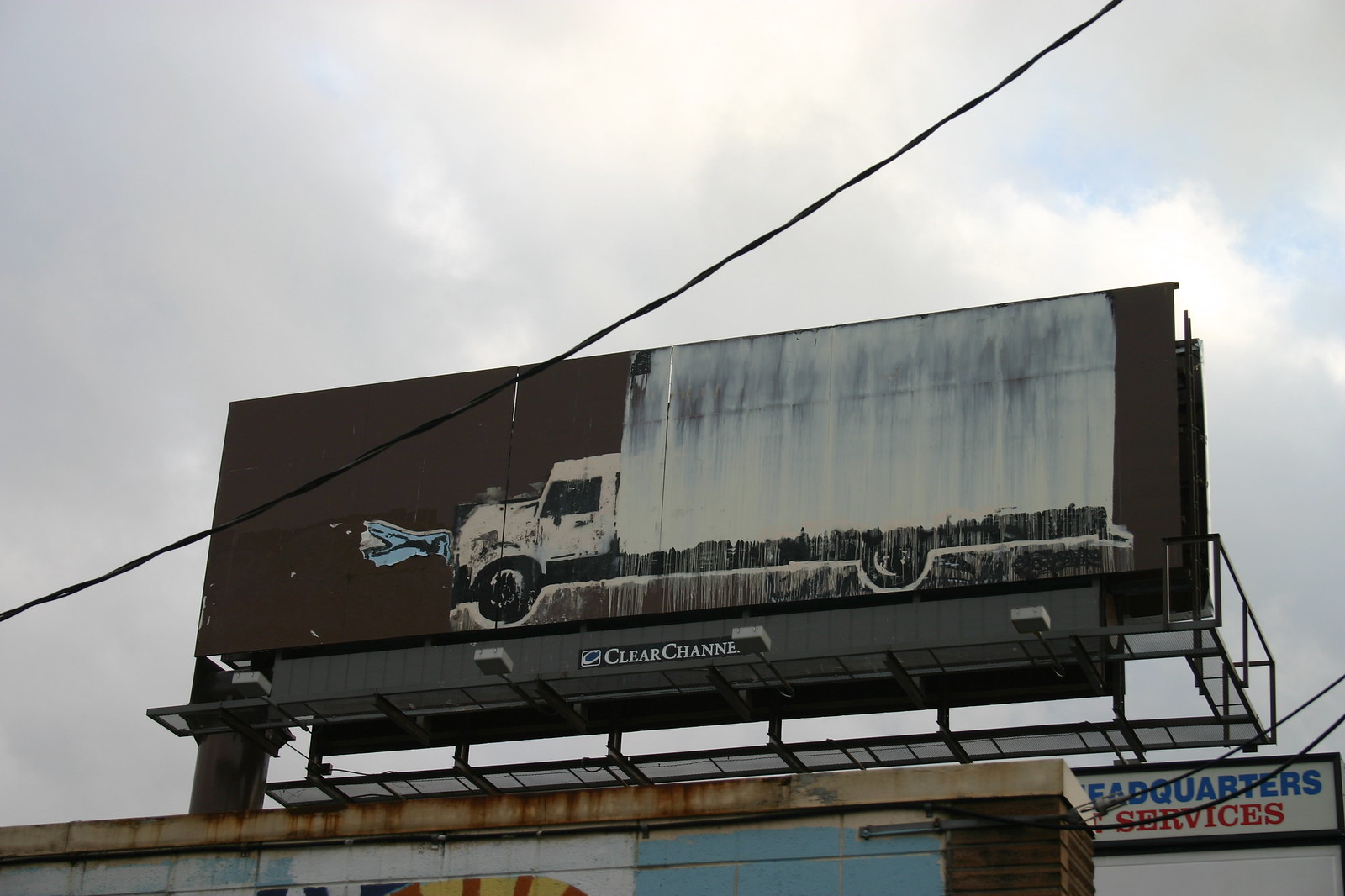This image depicts a billboard set against a heavily clouded sky with patches of blue, suggesting an impending rain. The billboard is mounted atop a rusted, white-painted building with teal siding. The building's flat cement roof and brick wall are partially visible at the bottom of the image. The billboard has a black frame and background, featuring a large white semi-truck with an ombre design transitioning from white to light blue, showing some transparency where the dark background peeks through. The truck is positioned as if traveling leftward (or in the 9 o'clock direction) with water spraying from its front. Below the truck image, there’s a gray rectangle that isn't as wide as the billboard, bearing a partially visible "Clear Channel" logo, though only "channel" can be read clearly. Square lights directed upwards are installed to illuminate the billboard at night. In the background, another building displays a partially visible sign reading "Headquarters Services" with "Headquarters" in blue and "Services" in red, though the "H" is cut off.